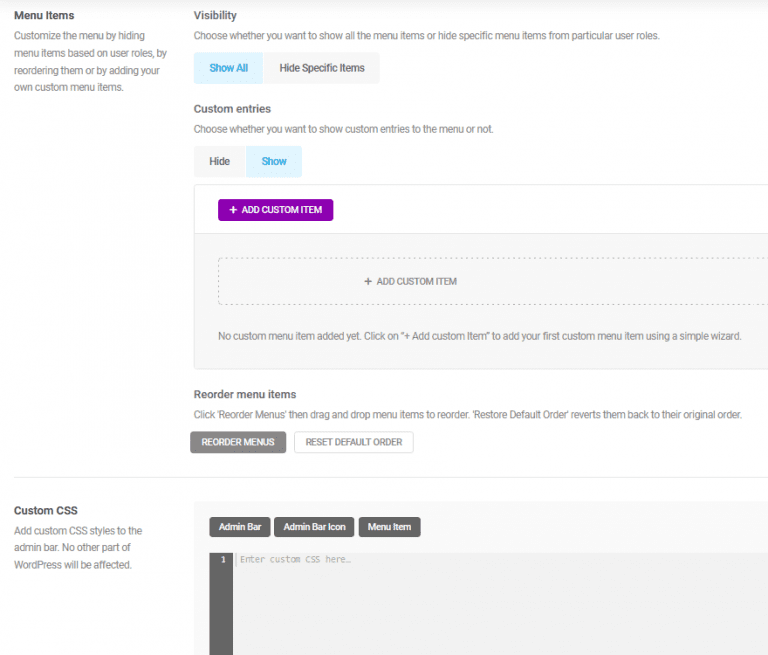This is a detailed screenshot of a website interface with a predominantly white background. The layout features text in various shades of gray, creating a visually stratified design. At the top left, there are bolded dark gray menu items, with supplemental information in lighter gray beneath them. Centrally, the image highlights customization options in medium gray text. The section on visibility is emphasized with bold text, accompanied by smaller light gray script. A notable bright blue "show all" option stands out, selected, with an adjacent "hide specific items" option.

The image also presents a fuchsia-colored, rectangular button in the center labeled "Add Custom Item" in white text. Beneath this button is a section designated for adding custom items, followed by a "reorder menu items" instruction. 

At the very bottom, three dark gray buttons offer additional functionalities labeled "Admin Bar," "Admin Bar Icon," and "Menu Item," each with white text for clear readability. This screenshot effectively conveys the hierarchical and functional design elements of the website’s customization interface.